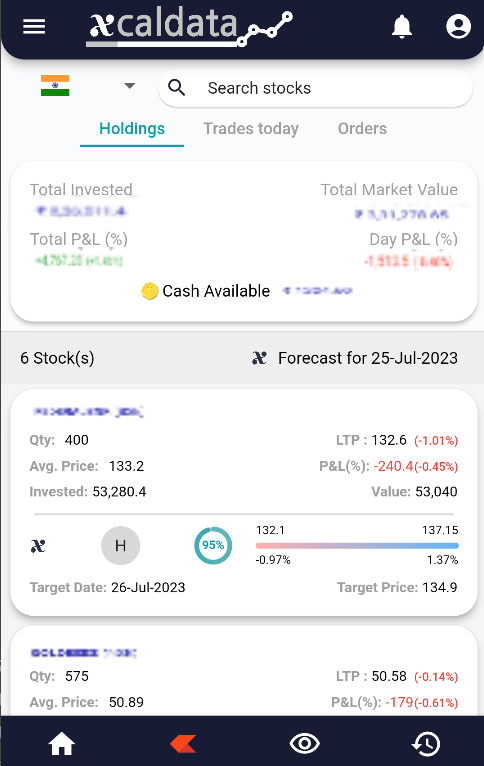**Detailed Screenshot Description of the XCalData App on a Mobile Device**

The screenshot captures the interface of the XCalData application on a mobile device. In the top right corner, there are icons for a notification bell and a small avatar. The three horizontal lines on the left indicate a menu option. Adjacent to these, a flag icon suggests an option to select the user's region or country, potentially altering the app's display settings.

Beneath these icons, a searchable interface is visible with a search bar labeled "Search Stocks" accompanied by a magnifying glass icon. The main menu below the search bar includes tabs labeled "Holdings," "Trades Today," and "Orders," with the "Holdings" tab actively selected.

Within the "Holdings" section, several data points are partially obscured. The upper part lists "Total Invested," "Total P&L Percent," "Total Market Value," and "Day P&L Percent," along with "Cash Available," all of which are blurred out.

The section below reveals detailed information about the user's stock portfolio. It shows holdings for six stocks with detailed metrics such as:
- **Date:** July 25th, 2023
- **Quantity:** 400
- **Average Price:** 133.2
- **Invested:** 53,280.4
- **LTP (Last Traded Price):** 132.6 (indicating a decrease of 1.01%)
- **P&L Percent:** -240.4 (a decline of 0.45%)
- **Value:** 53,040

Further down, a symbol marked with an "X" and an "H" within a gray circle is visible. A conspicuous green button labeled "95%" is also seen, likely indicating a confidence level in the given data.

Additionally, a "Target Date" is set for July 26th, 2023. This section includes a price range bar displaying values from 132.1 to 137.15, with a target price of 134.9. Underneath, further portfolio details include:
- **Quantity:** 575
- **Average Price:** 50.89
- **LTP:** 50.58 (a reduction of 0.14)
- **P&L Percent:** -179, equating to a -0.61% loss

This enriched and detailed description provides an articulate and comprehensive overview of the screenshot from the XCalData mobile application.